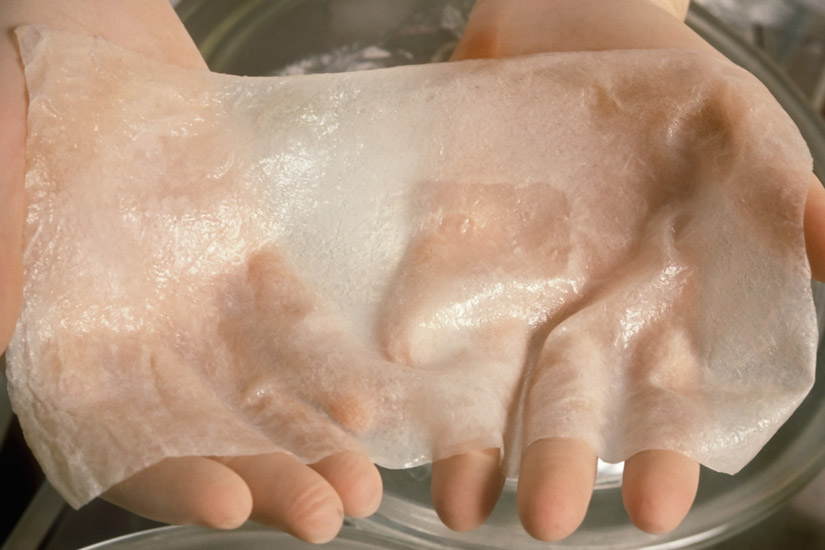In a close-up shot, two hands are seen holding a rectangular piece of artificial skin that closely resembles a wet paper towel. The hands prominently display the skin, which occupies almost the entire frame of the image. The skin appears whitish and slightly translucent, and its flexibility is evident from the subtle wrinkles, particularly noticeable on the right side. The lower part of the image reveals the fingers extending beneath the skin, while a portion of the arms is visible in the background, hinting at the flesh tone of the individuals handling the material. A shiny silver dish is situated underneath the piece of skin and the hands, suggesting that the scene is set in a laboratory environment. The artificial skin is meticulously handled, showcasing its pliability and texture.